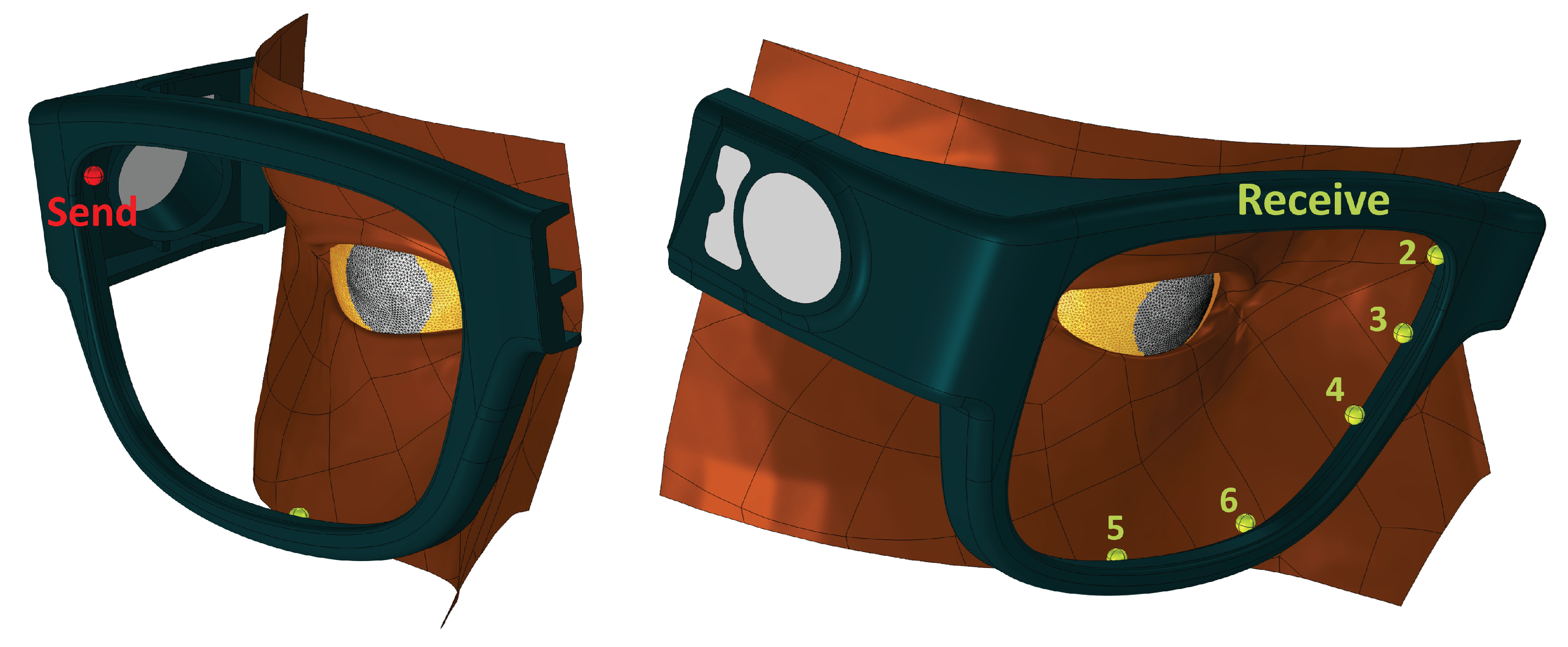The image is a detailed technical diagram illustrating high-tech glasses that communicate with a human eye. The background features a stylized golden eye with a black iris and no pupil, set against a brownish-bronze face. It consists of two main sections on a white backdrop. 

On the left, the diagram focuses on the mechanism for sending information. Here, you see the left side of the glasses, specifically highlighting the arm of the eyeglasses with a small red dot labeled "Send" near the joint where the arm meets the frame.

On the right, the diagram shifts to the receiving function. It showcases the same eye from a slightly different angle, revealing more of the face and part of the nose. The eyeglasses frame is lined with green points labeled 2, 3, 4, 5, and 6 along the midline edge, marked "Receive." There is a consistent black frame around the lenses in both sections, indicating the transmission and reception of information via these high-tech glasses.